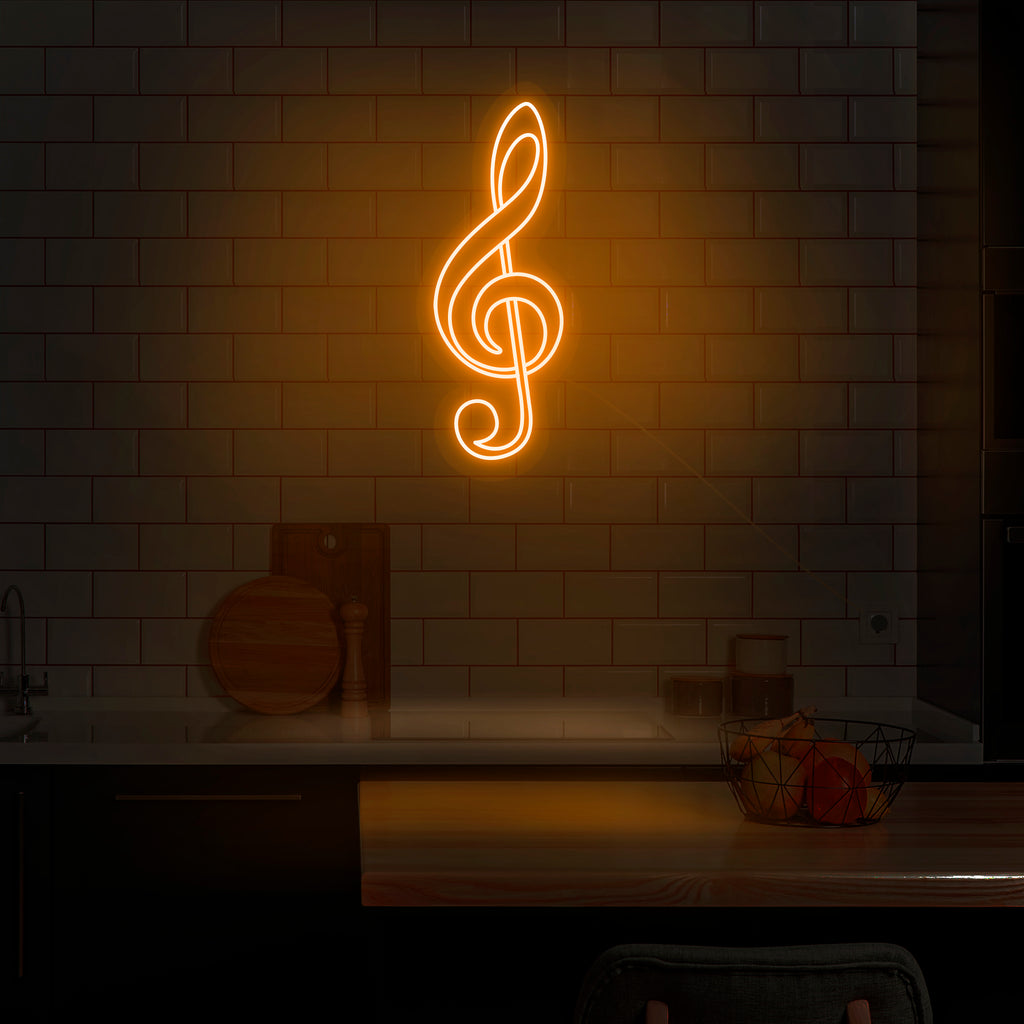The image shows a dimly lit room, likely part of an apartment, illuminated by a glowing neon treble clef symbol that hangs on a brick-designed wall. This treble clef emits a reddish, pinkish, orangish light, casting an ambient glow over the scene. The wall, appearing yellowish toward the center, retains a brick texture but fades to black along the edges. Beneath it, to the left, you can glimpse a white table that stretches across most of the image, on which a wooden cutting board and salt shaker rest. Nearby, two small green candles sit beside a white candle. Extending in front of this table is a glossy brown wooden table, adorned with a black basket containing various fruits like apples and oranges. A blue chair is partially visible in the bottom right corner, adding a pop of color to the otherwise dimly lit setting.